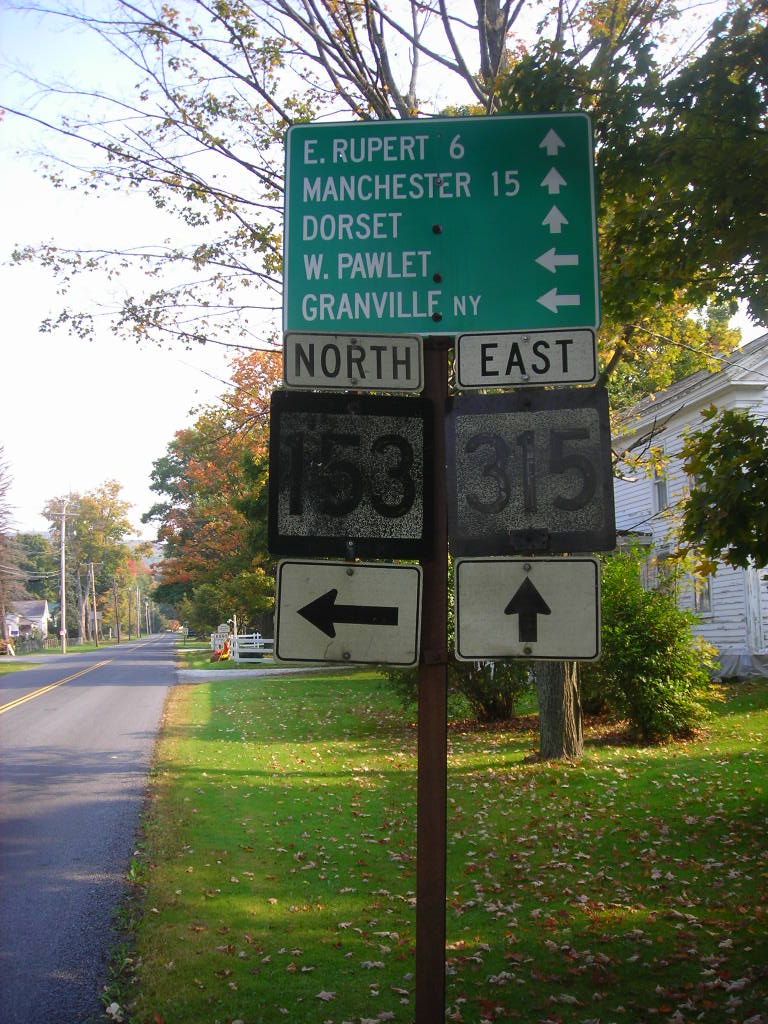The image showcases a tranquil rural scene. To the left, a winding road flanked by quaint houses and lush, distant trees leads the viewer's eye into the horizon. To the right, a vast expanse of verdant grass stretches out in front of a pristine white building, adding contrast to the picture. Dominating the foreground is a detailed road sign, indicating a junction ahead. The sign shows directions with numerical indicators: "153" pointing left and "315" pointing right, signifying north and east directions respectively. At the top of this sign, set against a backdrop of a majestic tree, is an additional green board with a white border. This sign lists the names of nearby towns in bold white capital letters, with some towns straight ahead and others indicating a left turn. The scene is bathed in natural light, highlighting the crisp details and serene atmosphere of this pastoral setting.